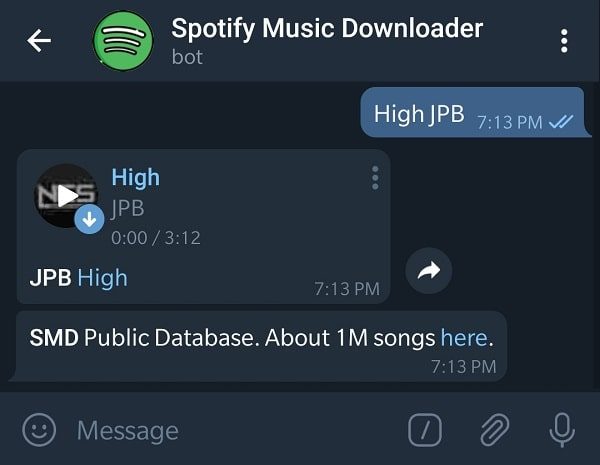This is a cropped screenshot of a mobile application interface. The screenshot features a dark bluish-gray header at the top. On the left side of the header, there is a white arrow pointing to the left. Adjacent to the arrow is a green logo outlined in black, featuring three slightly curved white lines that increase in size upward within the logo. To the right of the logo, the header displays white text that reads "Spotify Music Downloader." Beneath this text, on the left side, there is smaller white text reading "Bot." On the far right of the header, three white dots are stacked vertically.

Below the header, the interface shows a dark gray rectangle. In the top right corner of this section, there is a medium blue chat bubble with rounded corners, except for a small curved triangle on the bottom right side pointing to the right of the screen. Inside this bubble, white text reads "Hi JPB." Below and slightly to the right, light blue text shows the time "7:13pm," flanked by two stacked light blue checkmarks.

Further down, on the left side, there is a dark blue rectangle with rounded corners. Within this rectangle, white text in the bottom left reads "JPB." To the right, light blue text simply says "Hi." In the top left section of the rectangle, a black circle contains a white triangle pointing to the right. Some obscured white text appears behind this circle. Nearby, another light blue circle with a white arrow pointing downwards is visible. 

Above and to the right of this setup, thick light blue text spells out "Hi H-I-G-H." Below this text, medium gray text reads "JPB," followed by more medium gray text displaying "0:00 / 3:12," denoting a timestamp or playback duration.